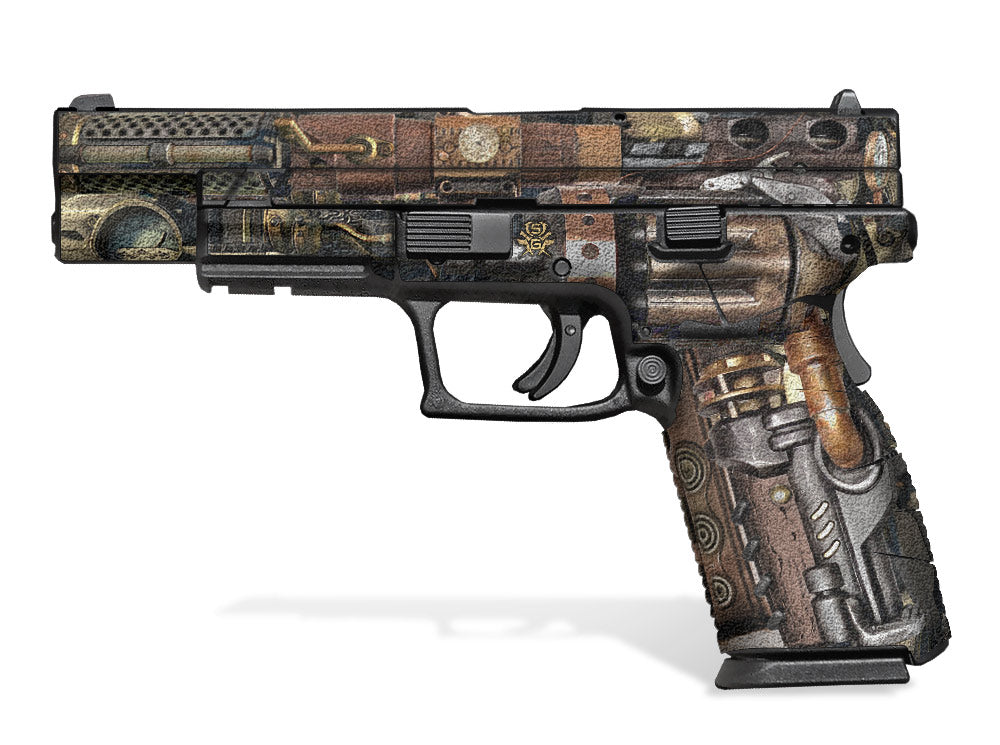The image depicts a highly detailed render of what appears to be a Glock 34 or 35 handgun, standing upright against a white background with a subtle drop shadow to its right. The firearm is oriented to the left and features a meticulously crafted steampunk-themed design. The intricate artwork spans almost the entire surface, except for the areas around the trigger and ammunition loading section, which remain black. This design is adorned with an array of mechanical elements such as pipes, venting areas, gears, and dials, painted in bronzes, browns, and golds, giving it an antique, industrial appearance. Noteworthy details include a prominent bronze-colored metal pipe illustration running along the back of the gun, a depiction of a clock, and even a flower motif. The artistic embellishments significantly enhance the aesthetic of the otherwise basic black pistol, making it look like an elaborate, mechanical masterpiece. This design resembles a skin that could be applied to the firearm, suggesting it may be an artistic render rather than a physical object.